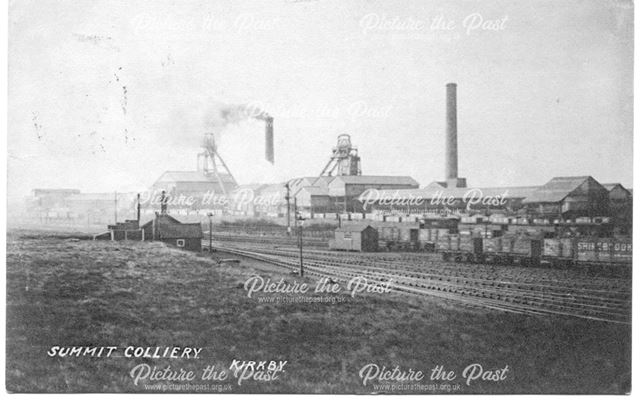This horizontally aligned, black-and-white postcard captures an old-time industrial scene, potentially of a series of factories or perhaps a coal power plant. Prominently featured are several rectangular buildings with two distinctive smokestacks, one actively emitting smoke. To the right, a line of railroad cars stands idle beside multiple railroad tracks. In the foreground lies a grassy area adjacent to the tracks, contrasting with the bustling, industrial background. Despite the complexity of structures depicted, the scene is notably devoid of people, imparting a desolate, bygone era atmosphere. The text “Summit Colliery” is printed at the bottom left, marking the location, and a repetitive watermark stating “picture the past” is scattered across the entire image, adding to its nostalgic significance. The sky appears light gray and cloudy, enhancing the vintage look of the photograph.